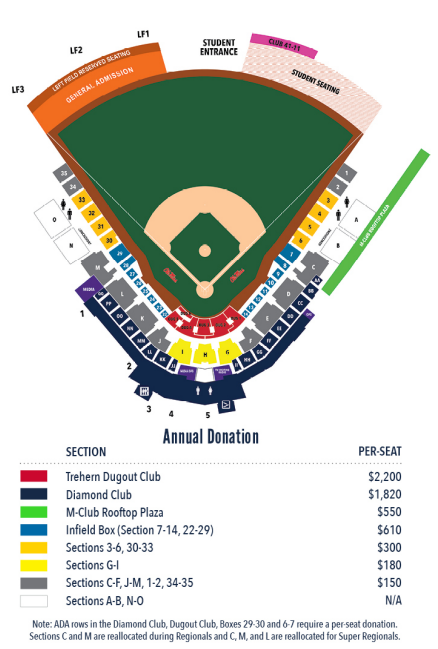A detailed top-down view of a professional baseball field, likely at a collegiate stadium, displays various seating arrangements and their corresponding donation requirements. The image features labeled areas such as the left field, right field, student seating, and general admission. Color-coded rectangles—red, black, green, blue, orange, yellow, gray, and white—indicate different sections including the Traehern Dugout Club, Diamond Club, M Club, Rooftop Plaza, and specific numbered sections.

These sections are designated as follows:
- Red: Traehern Dugout Club ($2,200 per seat)
- Black: Diamond Club ($1,820 per seat)
- Green: M Club ($550 per seat)
- Blue: Rooftop Plaza ($610 per seat)
- Orange: Infield Section 7-14 and 22-29 ($300 per seat)
- Yellow: Sections 3-6, 30-33 ($180 per seat)
- Gray: Sections G-I ($150 per seat)
- White: Sections C-F and J-M, 1-2, 34-35 (N/A per seat)
- Sections A-B and N-O (N/A per seat)

Additional details include ADA accessible rows in the Diamond Club Dugout Club (Boxes 29-30 and 6-7) which require a per seat donation. During regional and super regional games, sections C and M are relocated, with sections C, M, and L also relocated for super regionals. The "Annual Donation" mentioned suggests that the prices listed might be contributions required for season tickets.